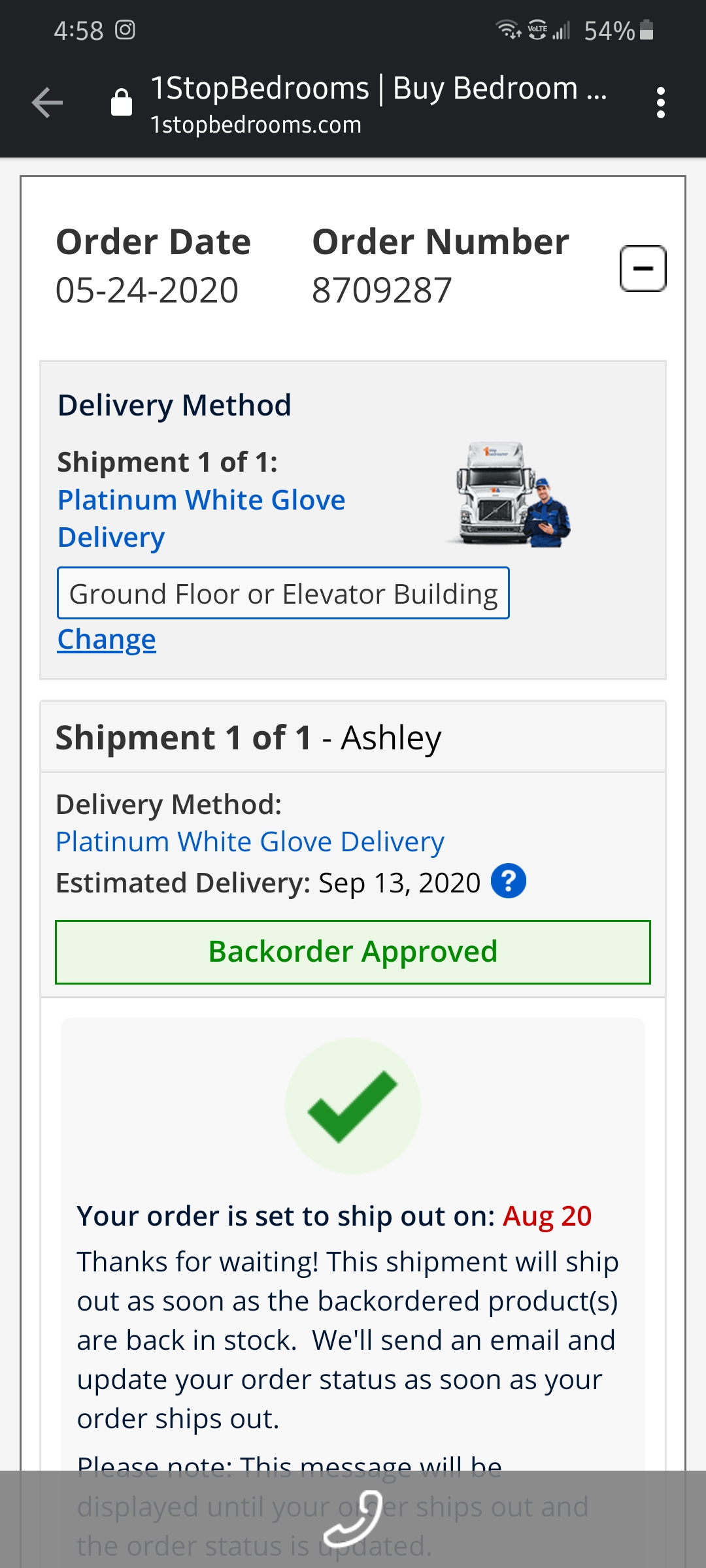Screenshot of an order page from "One Stop Bedrooms" on a mobile phone. The order page is displayed with black text on a white background. The order details show:

- **Order Date**: May 24, 2020
- **Order Number**: 870-9287

Below the order details, there are two rectangular sections with gray backgrounds labeled "Delivery Method":

1. **First Section**:
   - **Shipment Number**: 101
   - **Delivery Method**: Platinum White Glove Delivery
   - **Delivery Details**: Ground floor or elevator building
   - **Visuals**: An image of a truck with a delivery man standing in front of it

2. **Second Section**:
   - **Shipment Number**: 101 (Ashley)
   - **Delivery Method**: Platinum White Glove Delivery
   - **Estimated Delivery**: September 13, 2020

Additionally, there is a light green box with green text and a dark green border, indicating "Back Order Approved."